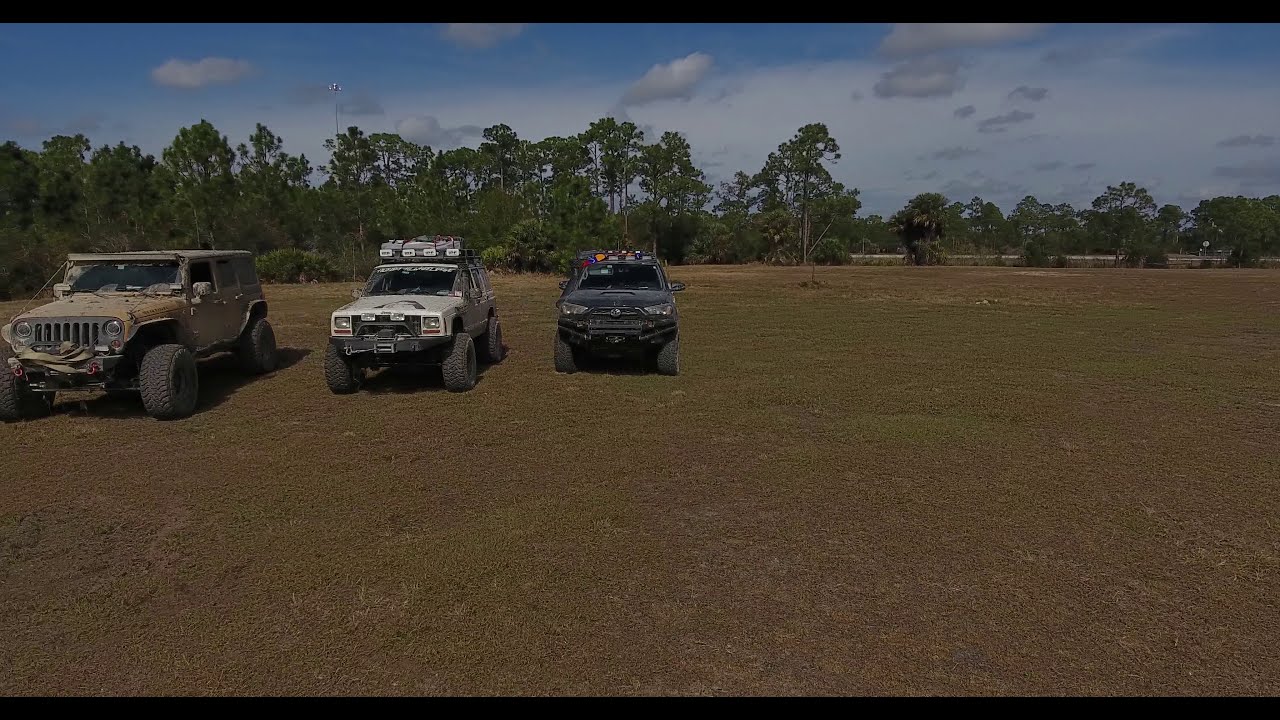In this photograph taken in a rural, dirt-filled field, three off-road vehicles are prominently lined up from left to right. The first vehicle on the left edge is a brown-colored Jeep, possibly just covered in mud and dirt. Next to it is a white truck, distinguished by bright lights mounted above its cab. The third vehicle, positioned centrally in the photo, is a darker-colored truck, potentially black or dark blue, also equipped with an array of lights on the roof. All three vehicles feature rugged, oversized tires. The field itself shows patches of green grass interspersed with significant areas of brown, suggesting dead grass or mud. Beyond the vehicles is a row of trees with a blue sky and scattered clouds overhead, and there appears to be a cell tower in the far distance.